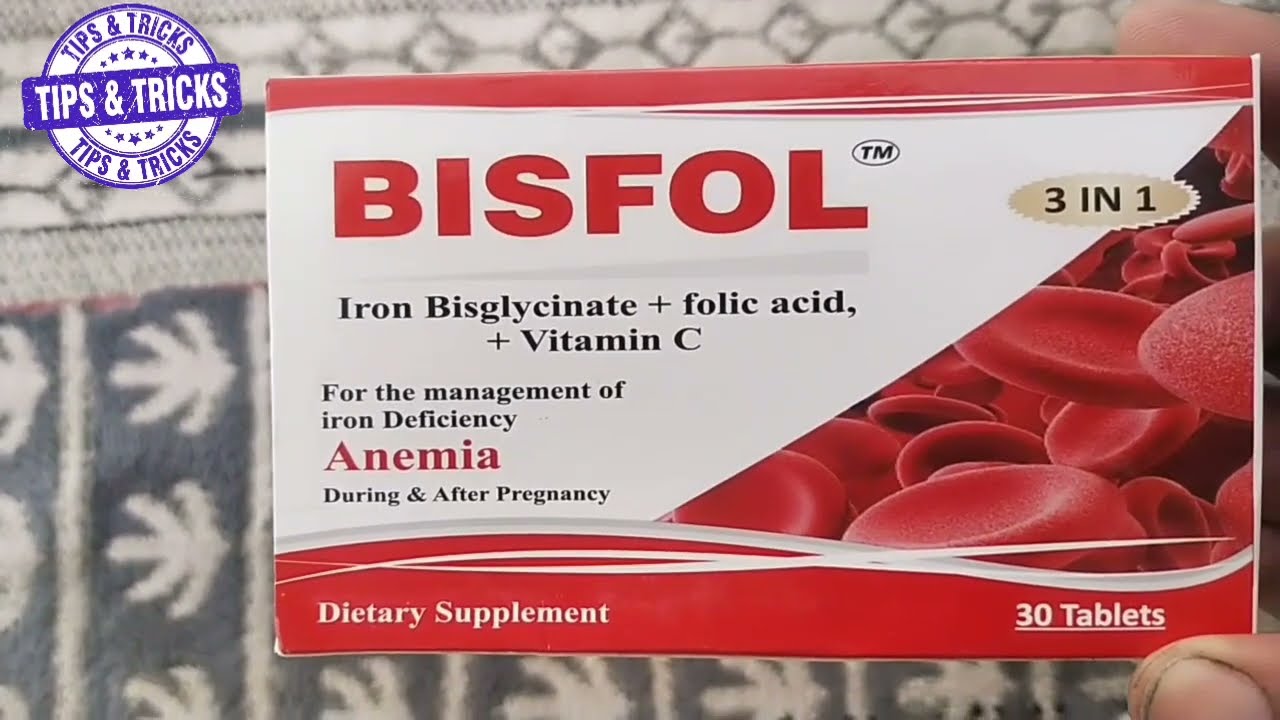The image showcases a close-up of a dietary supplement package held by someone's right hand with a dirty thumbnail. The package, set against a carpet background, is predominantly red and white. The top component is a bright red strip with a white strip below it. At the top left corner, there's a round purple seal with the text "Tips and Tricks" repeated thrice in a purple rectangle, surrounded by stars. The product name "BISFOL" is prominently displayed in red, with additional text indicating it is an iron bisglycinate plus folic acid and vitamin C supplement, intended for managing iron deficiency anemia during and after pregnancy. The package further notes that it is a 3-in-1 dietary supplement, containing 30 tablets. Red blood cells are illustrated on the right side of the package.